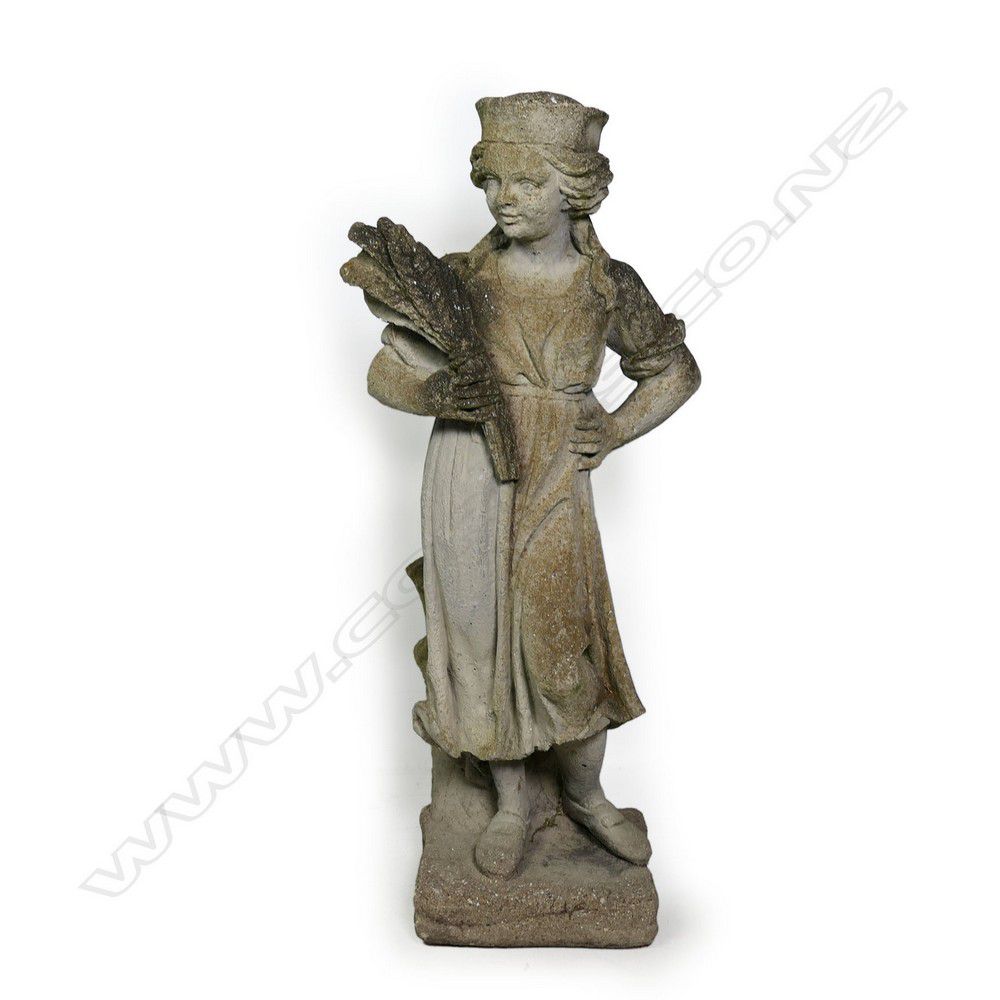The image depicts a weathered stone statue of a young woman, sourced from a stock photo service, evidenced by an indistinct watermark that stretches from the bottom left to the top right corner. The statue, carved from a beige whitish stone now marred by black, brown, and green discolorations, showcases signs of weathering, with darker moldy areas, chips, and an overall dirty appearance. The young woman is adorned in a cap and a simple cloth robe that falls to her mid-calf, revealing her sandaled feet, one of which is turned outward. In her right hand, she holds a bushel of produce, possibly sheaves of wheat or spiky flowers, resting on her shoulder, while her left hand is poised on her hip. She gazes to her left, standing on a small pedestal made of the same deteriorated material.